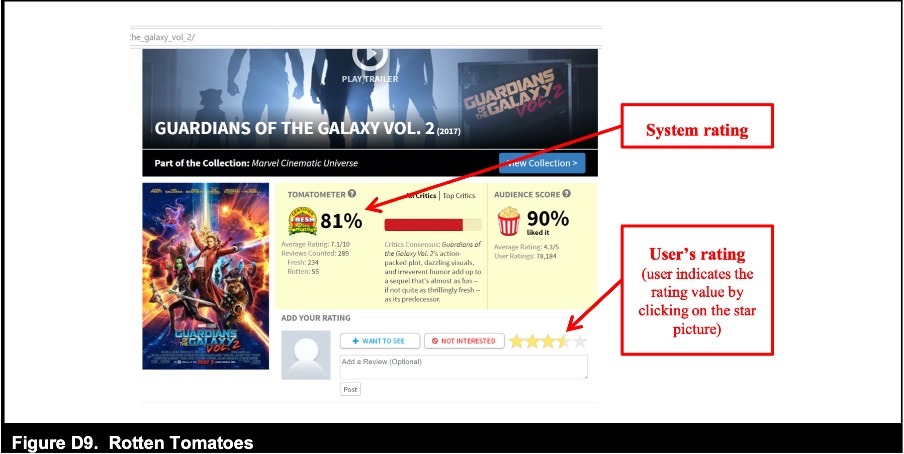This detailed image captures a screenshot of the Rotten Tomatoes website, labeled as Figure D9. It prominently features the page for the movie "Guardians of the Galaxy Vol. 2." At the top of the page, there is an embedded trailer for "Guardians of the Galaxy Vol. 2." Below the trailer, the Tomatometer is displayed, showing ratings and reviews from critics and the audience. On the right side of the screenshot, a highlighted rectangle has been drawn around the film's critic score, which stands at 81%. Additionally, a separate box highlights a star symbol representing the user rating for the movie.